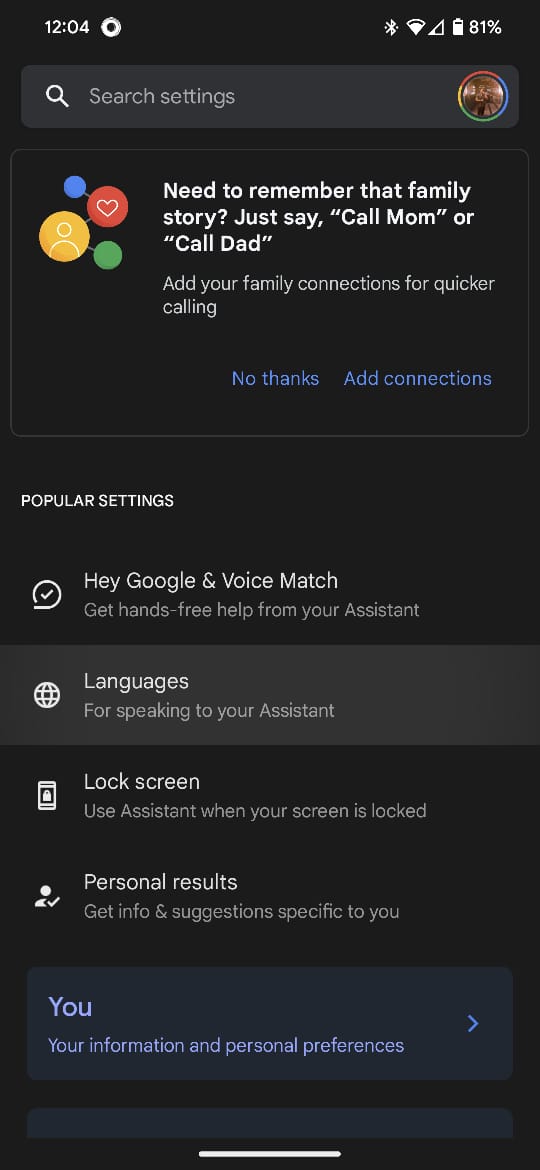The image is a screenshot taken from a mobile device. The background is black, and the top left corner displays the time "12:04" in white text, accompanied by an icon resembling a thick ring with a hole in the middle. On the top right corner, there are several status icons: the Bluetooth icon, the cellular signal strength icon, the Wi-Fi strength icon, and the battery percentage, which shows "81%". 

Below these indicators, there is a search bar featuring a magnifying glass icon with the text "Search settings". To the right of the search bar is a circular profile picture, encircled by a multicolored ring in shades of yellow, red, blue, and green.

Further down, the image displays an icon made up of four circles in blue, red, yellow, and green, each connected by lines. The yellow circle contains a drawing of a person, while the red circle has a heart symbol. Adjacent to this icon, text reads, "Need to remember that family story? Just say, 'Call Mom' or 'Call Dad'. Add your family connections for quicker calling". Below this message, there are two buttons: one labeled "No thanks" and the other "Add connections".

At the bottom of the screenshot is a list titled "Popular Settings," which includes the following options: "Hey Google & Voice Match," "Languages," "Lock Screen," "Personal Results," and finally, "Your information and personal preferences."